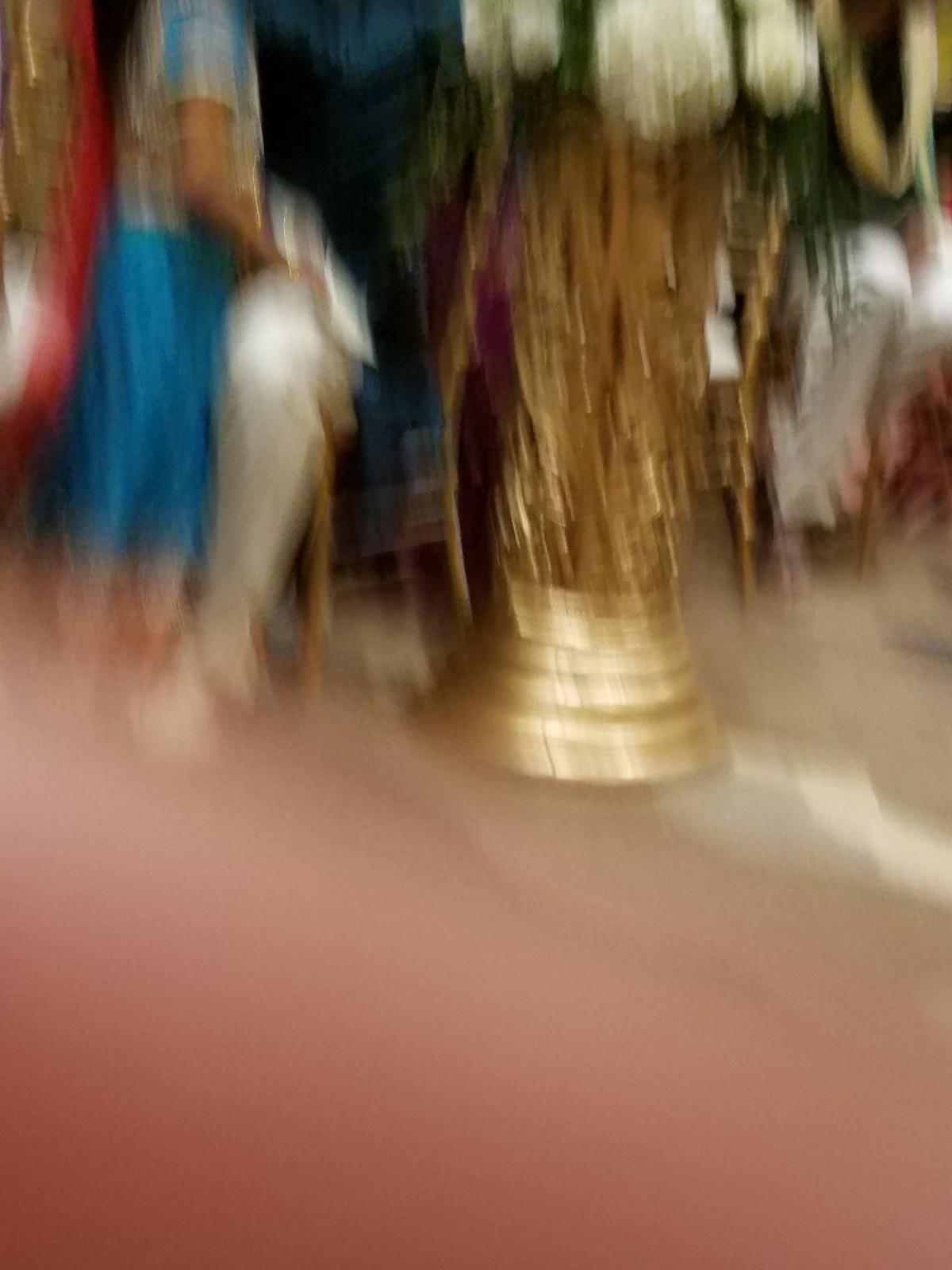A blurry, out-of-focus photograph partially obscured by a finger at the bottom, tinged with a pink, skin-toned color. The scene appears to be indoors, featuring a tan-colored floor. A woman stands prominently in the frame, dressed in a striking blue and gold dress, holding a white jacket or shawl in her hands. Behind her, there is what seems to be a gold, metallic statue or structure with ornate designs, though the lack of focus makes it difficult to ascertain its details. The overall composition creates a mysterious and somewhat abstract visual narrative due to its unintended obstructions and blurred elements.